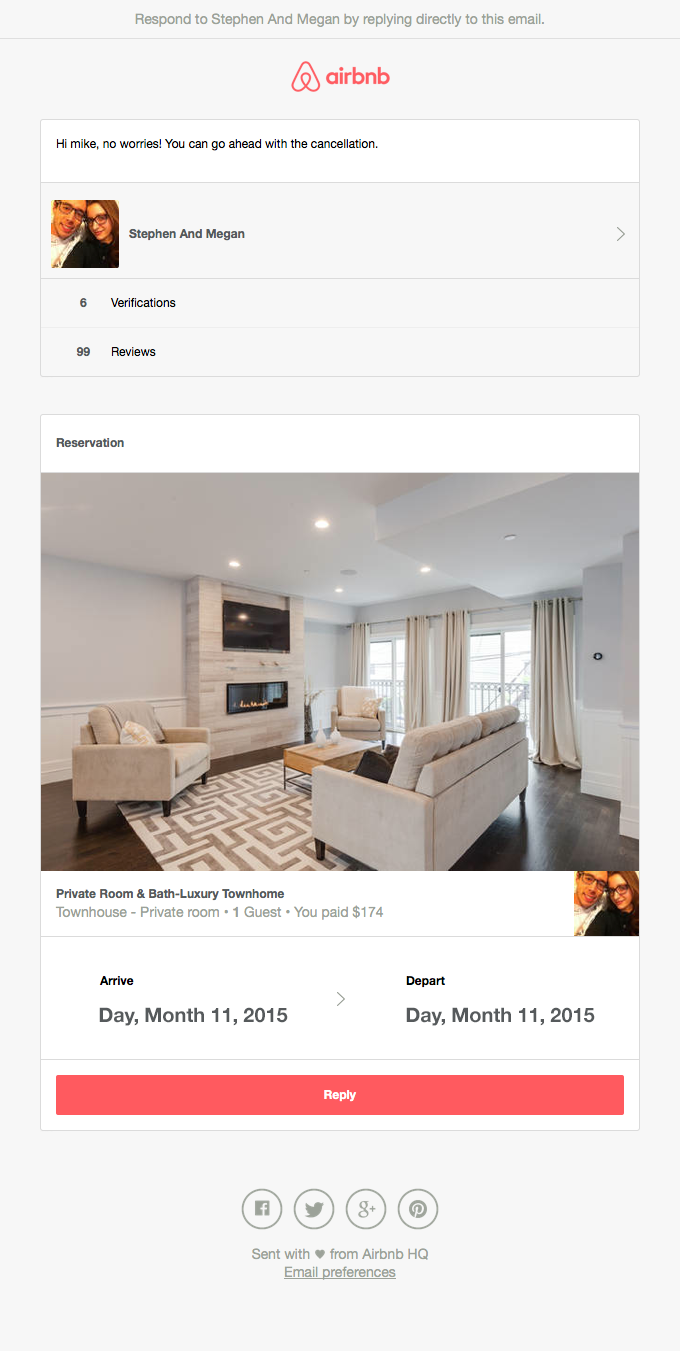This image is a screenshot from the Airbnb website, displaying a message received by a user named Mike. At the upper center of the message, light gray text provides instructions: "Respond to Steven and Megan by replying directly to this email." Below this guidance, the Airbnb logo is prominently centered on the screen.

In a central white rectangular box, the message from the hosts reads: "Hi Mike, no worries, you can go ahead with the cancellation." To the left of this message, there is an image of a smiling couple, both wearing dark-colored glasses. The individuals are identified by the text "Steven and Megan" positioned to the right of their picture.

Additionally, there are six verifications listed beneath their names, alongside the text indicating that their listing has garnered "99 views." Further down, a smaller box displays an image of a living room in an apartment, which is related to the reservation.

The listing is titled "Private Room and Bath, Luxury Townhome," described in further detail as "Townhouse, private room, one guest." The cost of the booking is mentioned: “You paid $174.” Adjacent to these details is another picture of Steven and Megan.

Finally, the arrival and departure dates are noted, both falling in November 2015. At the very bottom, a prominent pink call-to-action button labeled "Reply" invites the user to respond to the message.